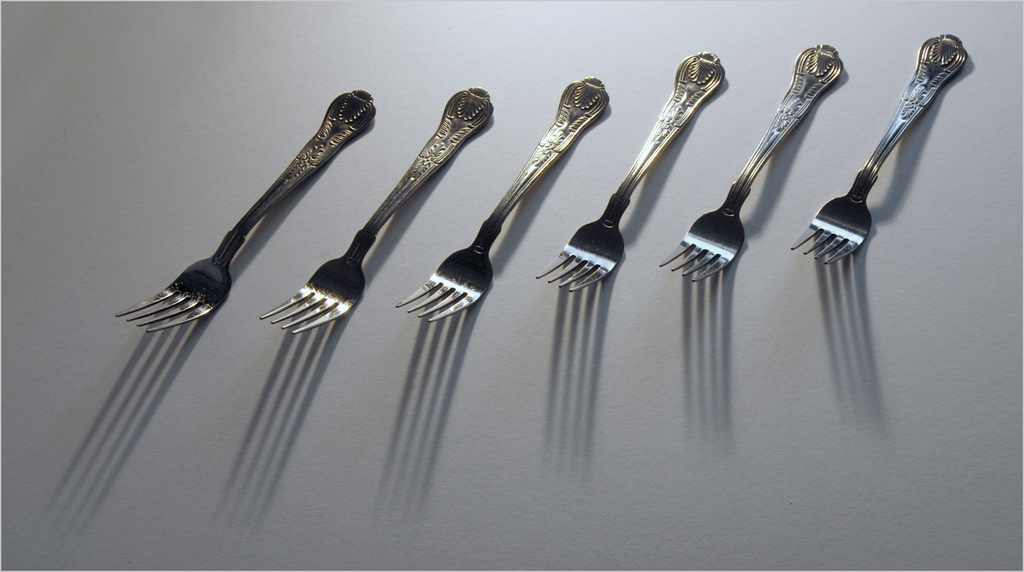The indoor color photograph depicts a collection of six silver forks aligned in a row against a primarily white background that subtly transitions to gray on the left and right edges. The forks are arranged diagonally, with their handles pointing towards the upper right and their prongs towards the lower left. The light source, positioned above, casts shadows directly beneath the prongs of each fork, which extend downward. Each fork is identical, featuring rounded tops with subtle silver indentations for design, and they are equidistantly spaced about an inch apart. The forks are positioned in such a way that each successive fork is slightly higher than the previous one, creating a slight upward diagonal ascent. The pristine, reflective quality of the forks and the interplay of light and shadow on the background accentuate the simplicity and elegance of the scene.